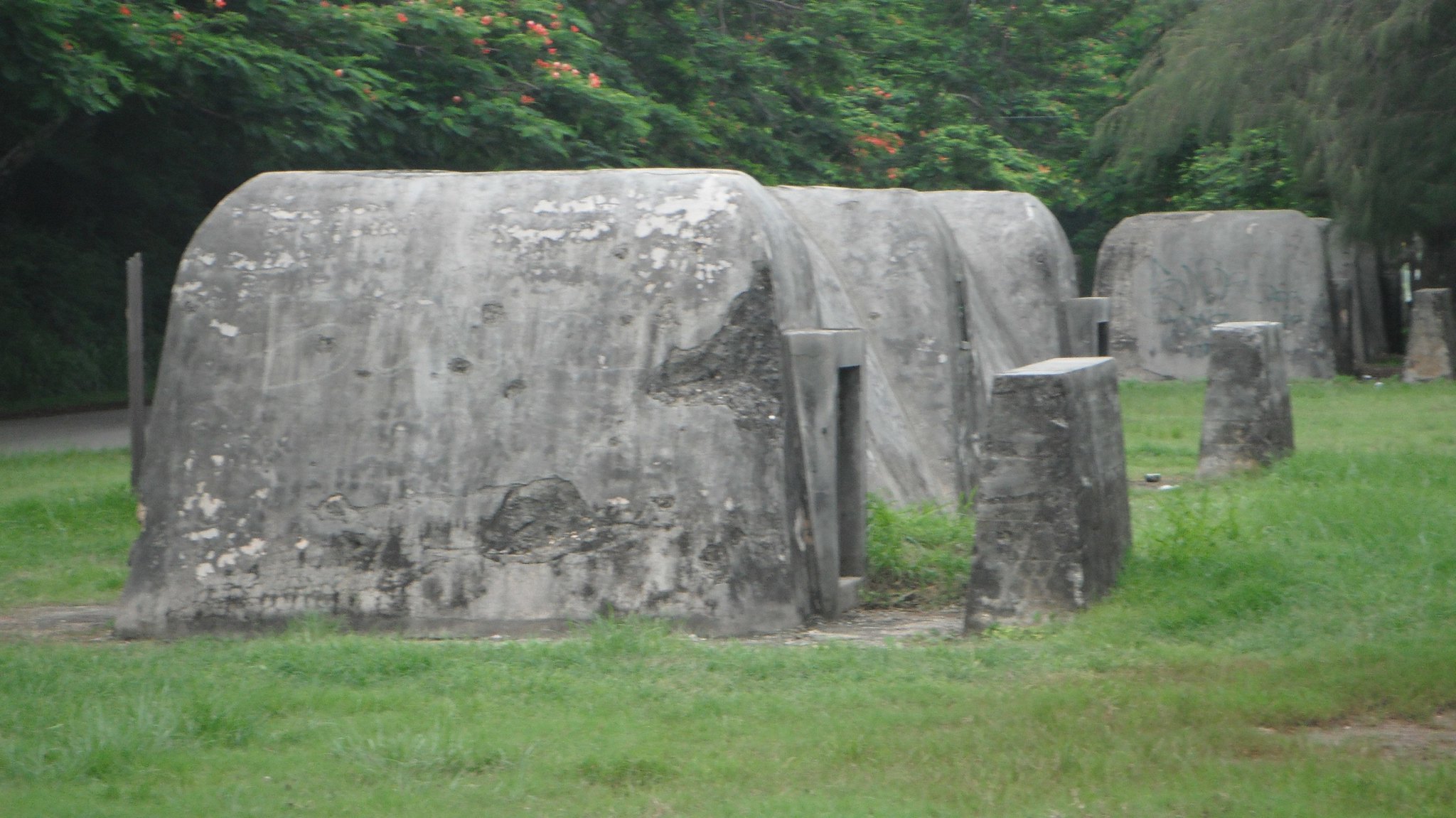Amidst a lush, green grassy field with dense, leafy trees in the background, there are four intriguing, man-made structures arranged in a row. These structures, resembling large oblong igloos or rounded huts made from concrete, exhibit weathered shades of gray, black, and white, with some areas showing signs of peeling paint. Each structure features a small, square entrance framed with stone, creating an impression of a doorway. Positioned directly in front of two of these huts are dark, headstone-like slabs, possibly made of marble, standing upright as if to mark or identify the structures. Shadows cast by the trees on the left side add depth to the scene, while patches of dirt around the entrances contrast with the vibrant, blush-green grass covering the ground. The scene is serene, yet the mysterious, tomb-like huts invite curiosity about their purpose and origin.